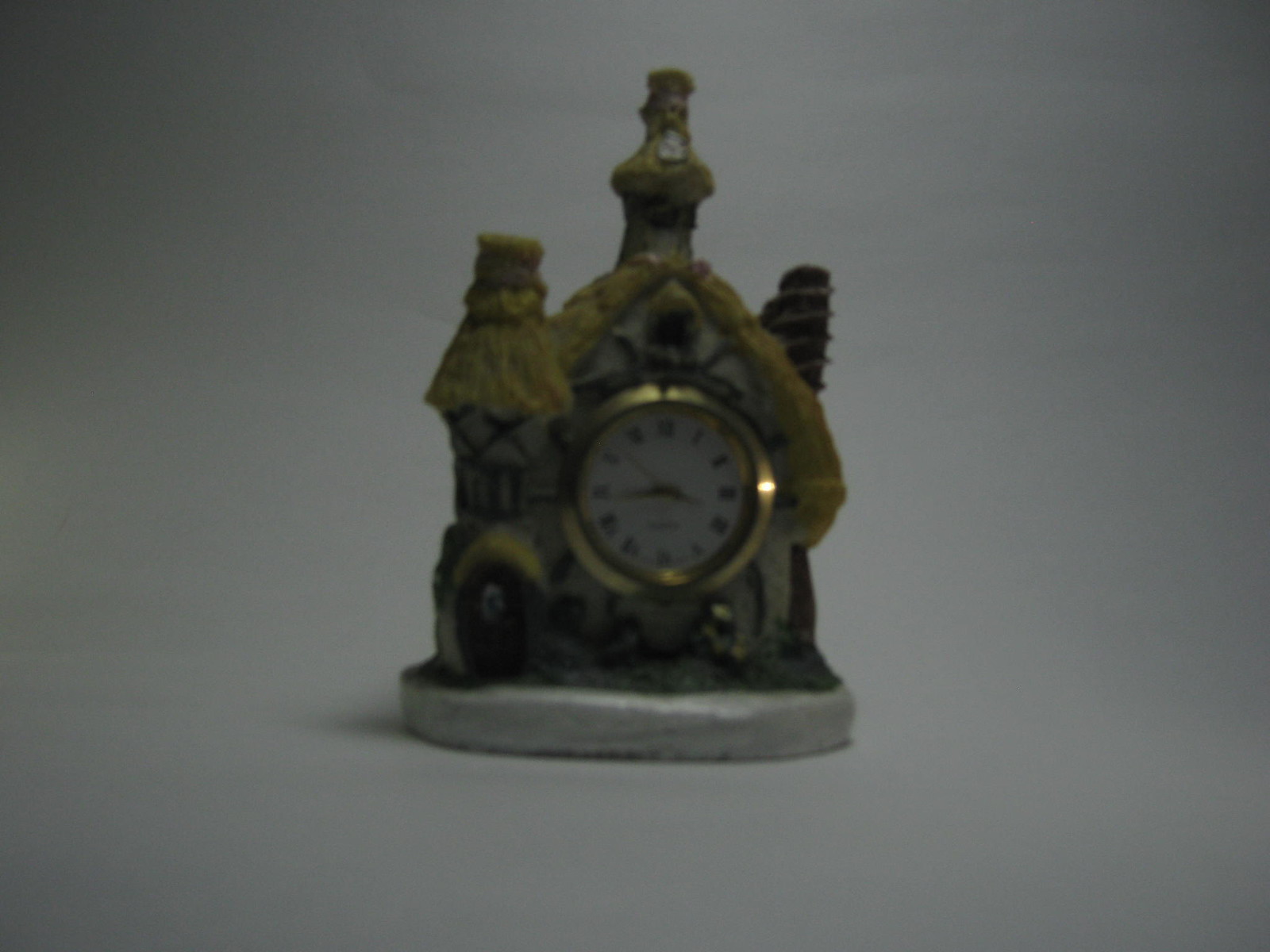This is a detailed photograph of a charming tabletop clock designed in the shape of a miniature medieval house or castle, set against a plain white backdrop that extends to the surface it sits on. The clock is not mounted on a wall but stands freely like a figurine, featuring a silver circular base. On this base sits a medieval-style house, adorned with a yellow straw hay roof that has multiple points. The roof has three protrusions on top, one possibly resembling a bearded man, adding to the intricate detail. 

The front of the house, where the clock face is located, is white with some green striping, and it features an arched wooden doorway positioned on the left. The clock itself, housed behind glass, has a white background with a gold border around it. It displays numbers 1 through 12 in black text alongside Roman numerals. The clock hands include a thinner minute hand, a shorter hour hand, and possibly a second hand, though that detail is blurred. The current time reads around 3:44, with the second hand near the 8-second mark. The overall design gives the impression of a quaint, detailed miniature castle clock.